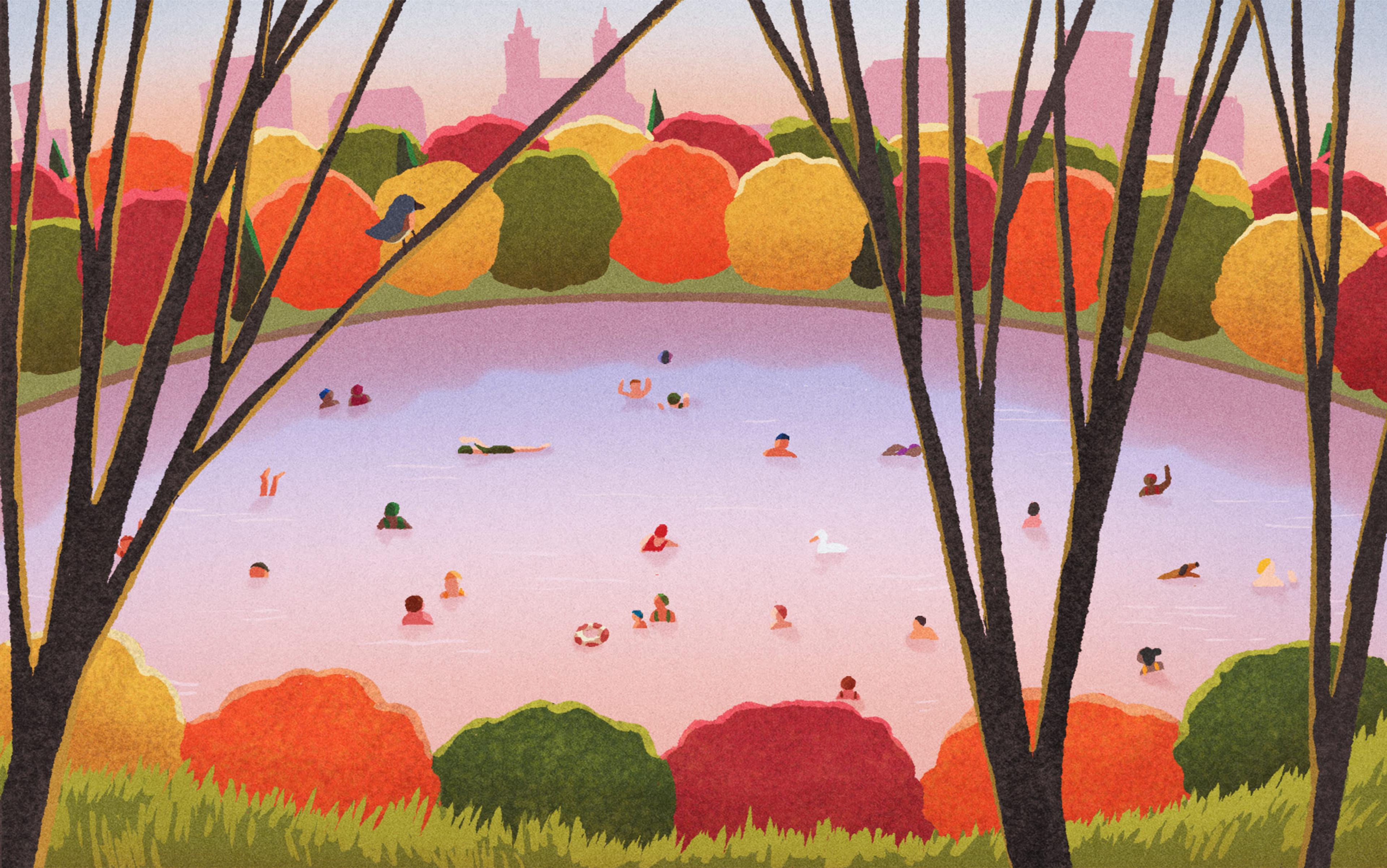The image is a vibrant, colorful painting depicting an animated scene of many people swimming in a large pool. The water, a blend of milky light blue, orange, and dark pink hues, reflects both the lively activity of the swimmers and the surrounding elements. The pool is defined by a thin, light brown curved edge. Scattered throughout the water, people are playing, with some engaging in ball games, creating an energetic and joyful atmosphere.

In the background, there are abstract clusters of multicolored foliage with hues of orange, dark green, yellow, and red, representing trees. These tree-like forms arch both above and below the central scene, framing the pool. Interspersed among them are green grassy patches that stretch horizontally across the bottom part of the scene. Emerging through the water and landscape, three prominently positioned brown tree trunks extend vertically—two on the right and one on the left—providing a sense of depth and layering.

Above this lively scene, the skyline showcases a pink silhouette of buildings against a backdrop of a light blue sky tinged with pink, adding a dreamy, almost surreal quality to the painting.